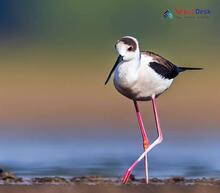In this outdoor photograph, a bird reminiscent of a kingfisher or stork stands prominently in the center with striking clarity. It is depicted with long, pinkish-red legs and a lengthy, slender black beak. Its plumage features a mix of colors: predominantly white on the breast and face, brown on the top of the head and back, and black on the wings, with a mostly black tail. The bird is positioned on a dark, muddy shoreline, possibly searching for food, facing towards the left side of the image. The background transitions from a dark, muddy ground at the very bottom to a blue hue that fades into orange and then green higher up, all appearing blurred. This suggests the scene is near a body of water under sunlight, enhancing the natural ambiance. In the upper right corner of the photo, there is a small, hard-to-read red and blue label, possibly containing the word "desk" and accompanied by a turquoise icon, potentially a globe. The image captures a tranquil, natural setting with the bird as the clear focal point, surrounded by the softly blurred colors of the outdoors.